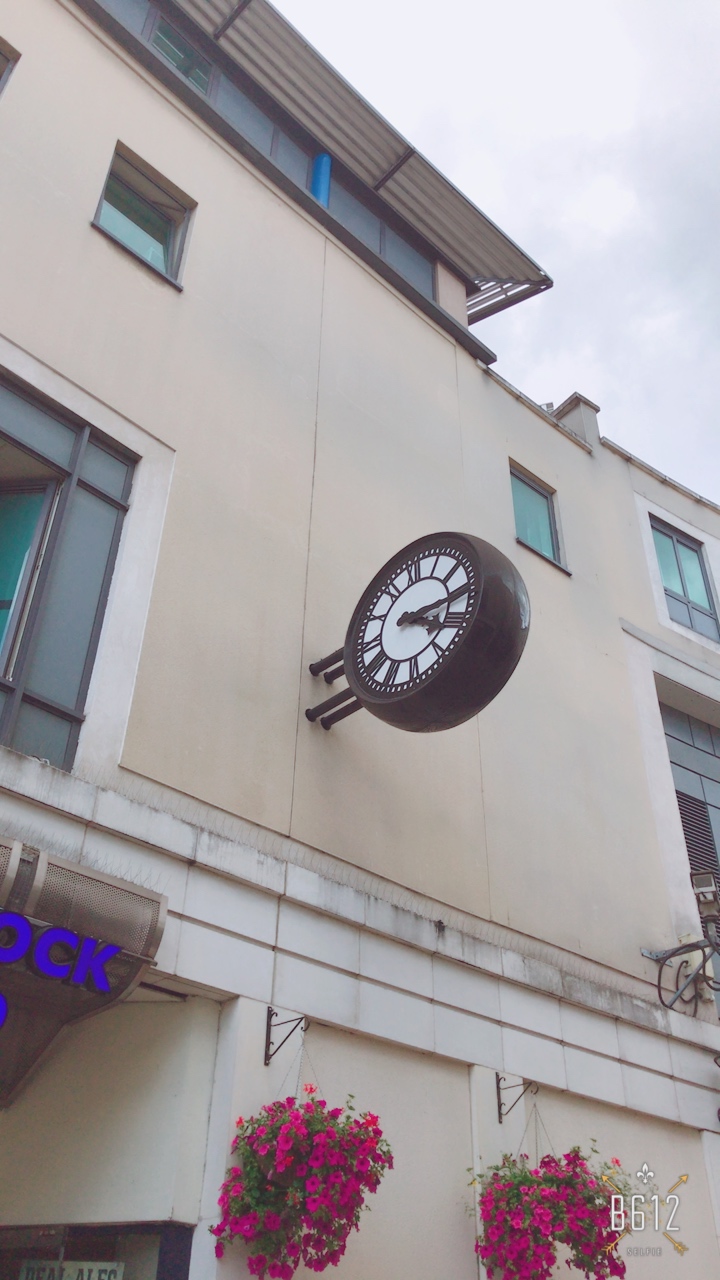This rectangular, horizontally-oriented photograph captures the exterior of a charming, two-story building. In the lower left part of the image, the entranceway is visible, subtly inviting exploration. Flanking the entrance on the right, two vibrant pots of hot pink flowers hang gracefully from the ceiling, adding a touch of lively color. Mounted on the exterior of the second floor, a striking clock juts out on decorative hardware. The clock features a black casing with a white face and black Roman numerals, with matching black hands to indicate the time. Above the entrance door, three large blue letters spell out "OCK," although other letters are not visible. In the lower right corner of the photograph, a watermark reading "B-612" is faintly stamped, marking the photograph’s source.